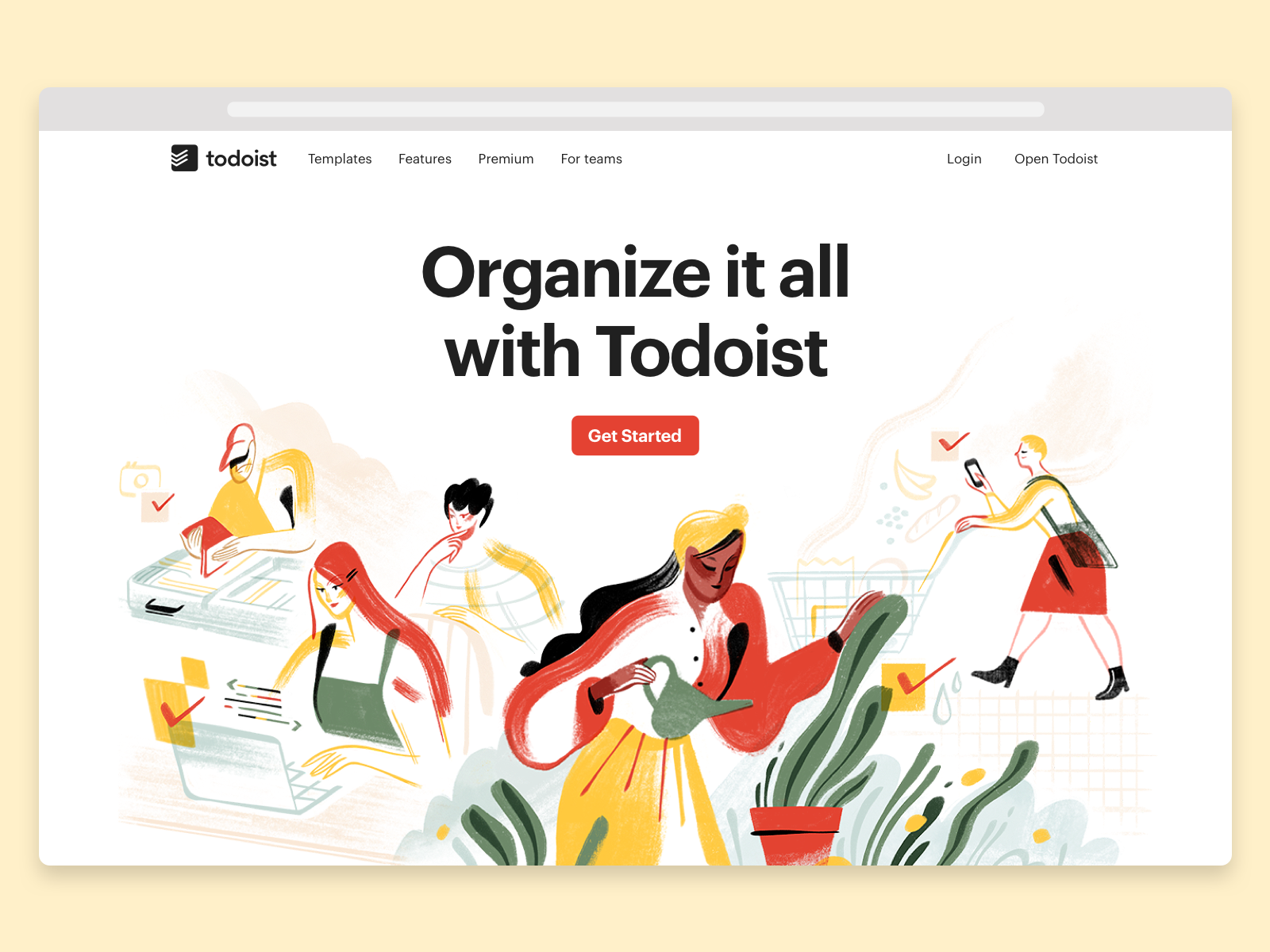The image depicts a polished web browser mock-up resembling familiar interfaces like Safari or Google Chrome. Displayed within this mock-up is a web page for Todoist, featuring its recognizable logo—a square with three stacked vertical lines resembling half chevrons. The header includes navigation options: "Templates," "Features," "Premium," and "For Teams," with "Login" and "Open Todoist" situated on the far right.

Dominating the middle of the screen is a prominent hero section bearing the bold text, "Organize it all with Todoist." Below this headline is a striking red button with white lettering that reads "Get Started." The background illustration is vivid and engaging, depicting people engaged with their computers and phones, as well as tending to a plant. The illustration employs a vibrant palette of red, yellow, black, and green, resembling a watercolor painting in its style and execution.